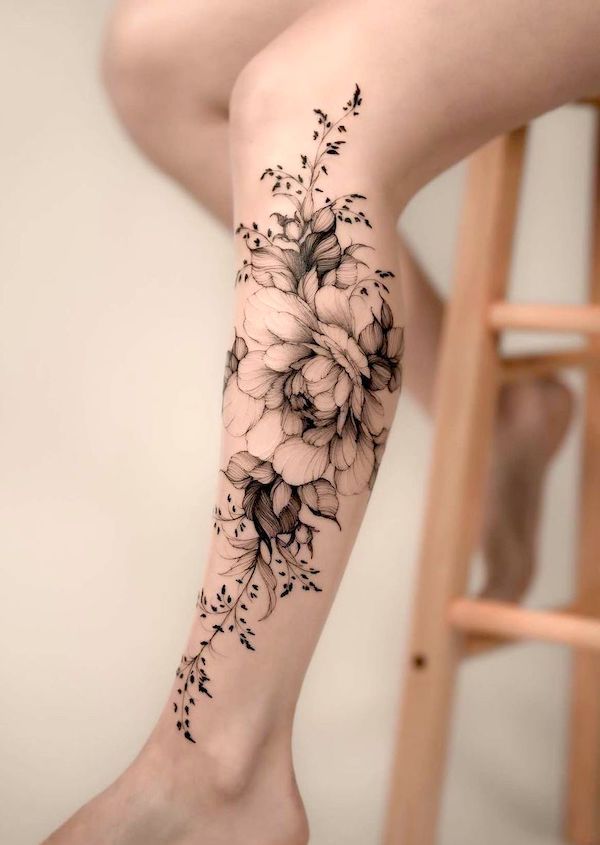The photograph depicts a Caucasian woman’s legs, adorned with a striking and intricate black and white floral tattoo. She is seated on a light wooden stool, with the white background creating a clean, minimalist scene. The detailed tattoo extends from just above her knee down to her ankle, featuring numerous petals and sprigs with tiny seeds, creating a vine-like appearance. Her left leg is primarily visible, showing the exquisite tattoo work, while her right leg is casually positioned on one of the stool’s supports. Only her legs, part of her feet, and the stool are visible in the image, with her feet partially blurred and cut off at the edges of the photograph. The main colors in the image are white, tan, and black, lending it a monochromatic and elegant aesthetic.